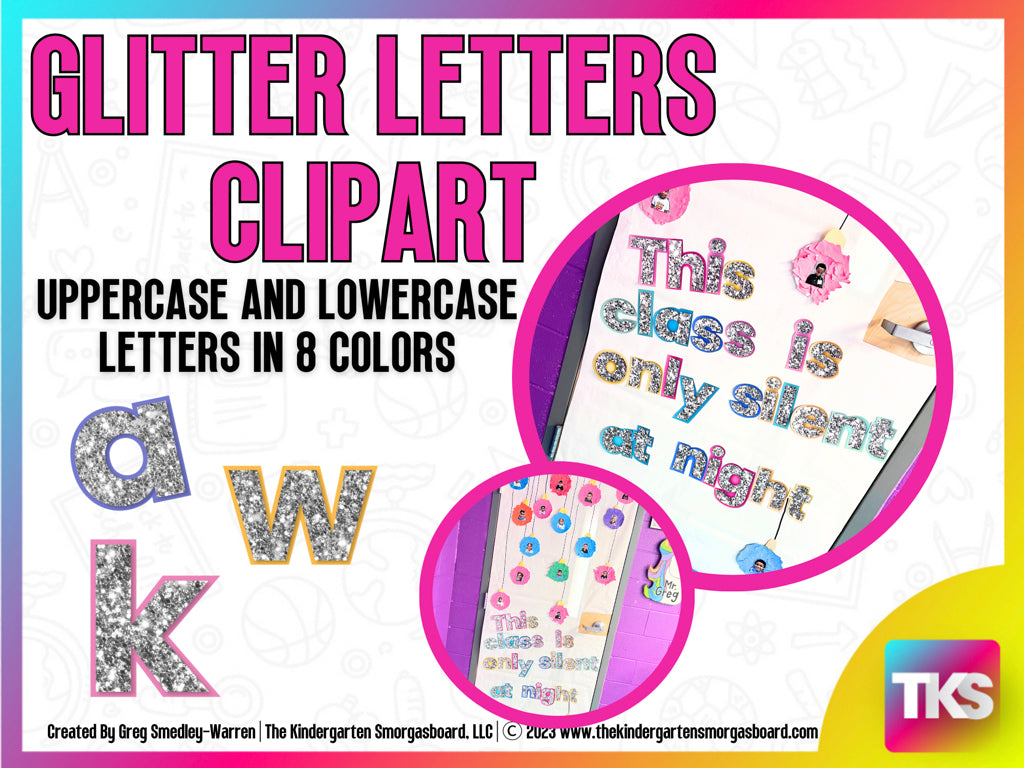This advertisement showcases glitter letters clip art with a vivid rainbow ombre border transitioning through colors: blue, purple, pink, orange, and yellow. In the upper left corner, the bold, capitalized font reads "GLITTER LETTERS CLIP ART," followed underneath by the assertion in black uppercase letters, "UPPERCASE AND LOWERCASE LETTERS IN EIGHT COLORS." Displayed in the lower left corner are example glittery letters "a," "w," and "k" in silver glitter. Dominating the right side of the image, two circular overlays present the phrase "This class is only silent at night" in the same glittery letters— the top circle larger and the bottom circle smaller. Finally, the lower right corner contains a distinctive rainbow square with "TKS" inscribed in white font, concluding the vibrant and engaging presentation.